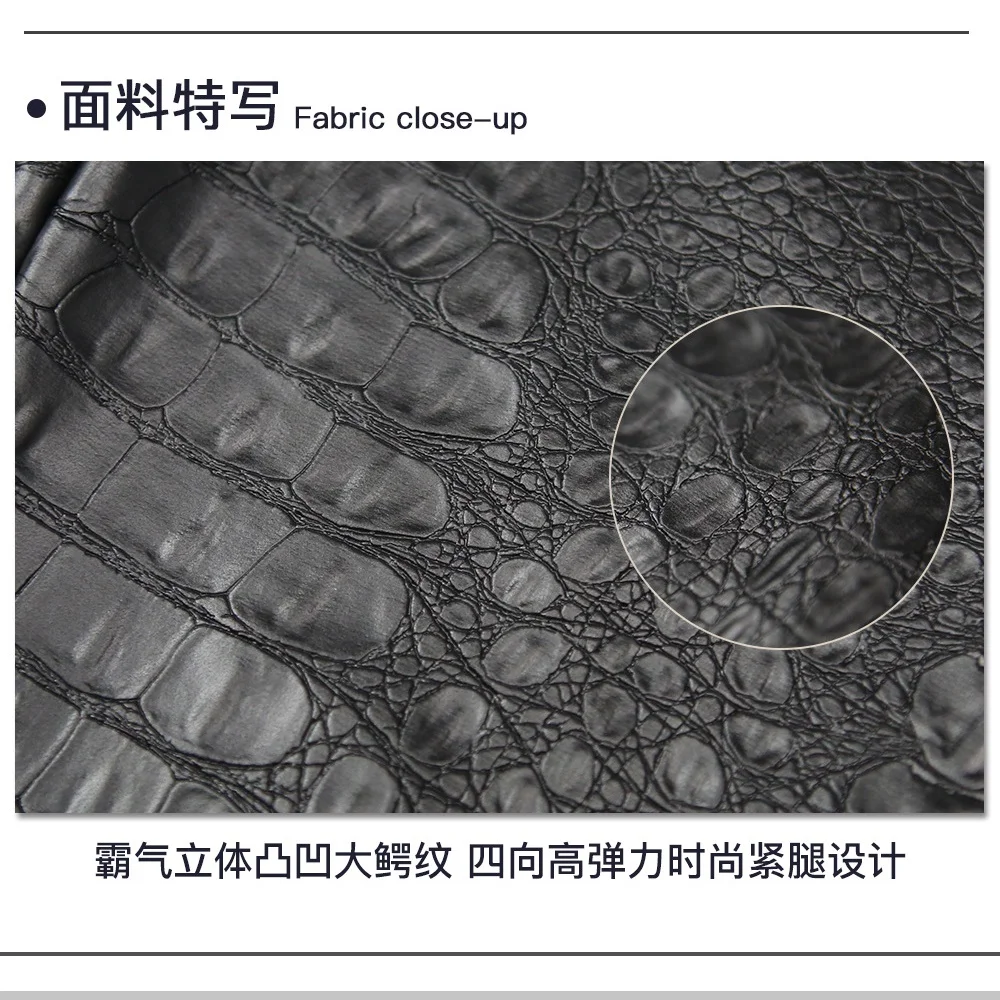The image appears to be a detailed textbook illustration related to textiles or fashion design, and it's primarily rendered in black and white. The central focus is a microscopic close-up of some type of fabric, with the only English text being the phrase "fabric close-up." The legend accompanying the image is predominantly in an Asian language, likely Japanese or Chinese. The highlighted section within a white circle shows the intricate textures of the fibers, which exhibit a pebbled and wrinkled appearance, closely akin to leather or vinyl. Additionally, there are aligned rectangular and square shapes on the left side of the image, resembling the segments of fingers, which might suggest that this fabric is potentially being prepared for the manufacture of gloves.